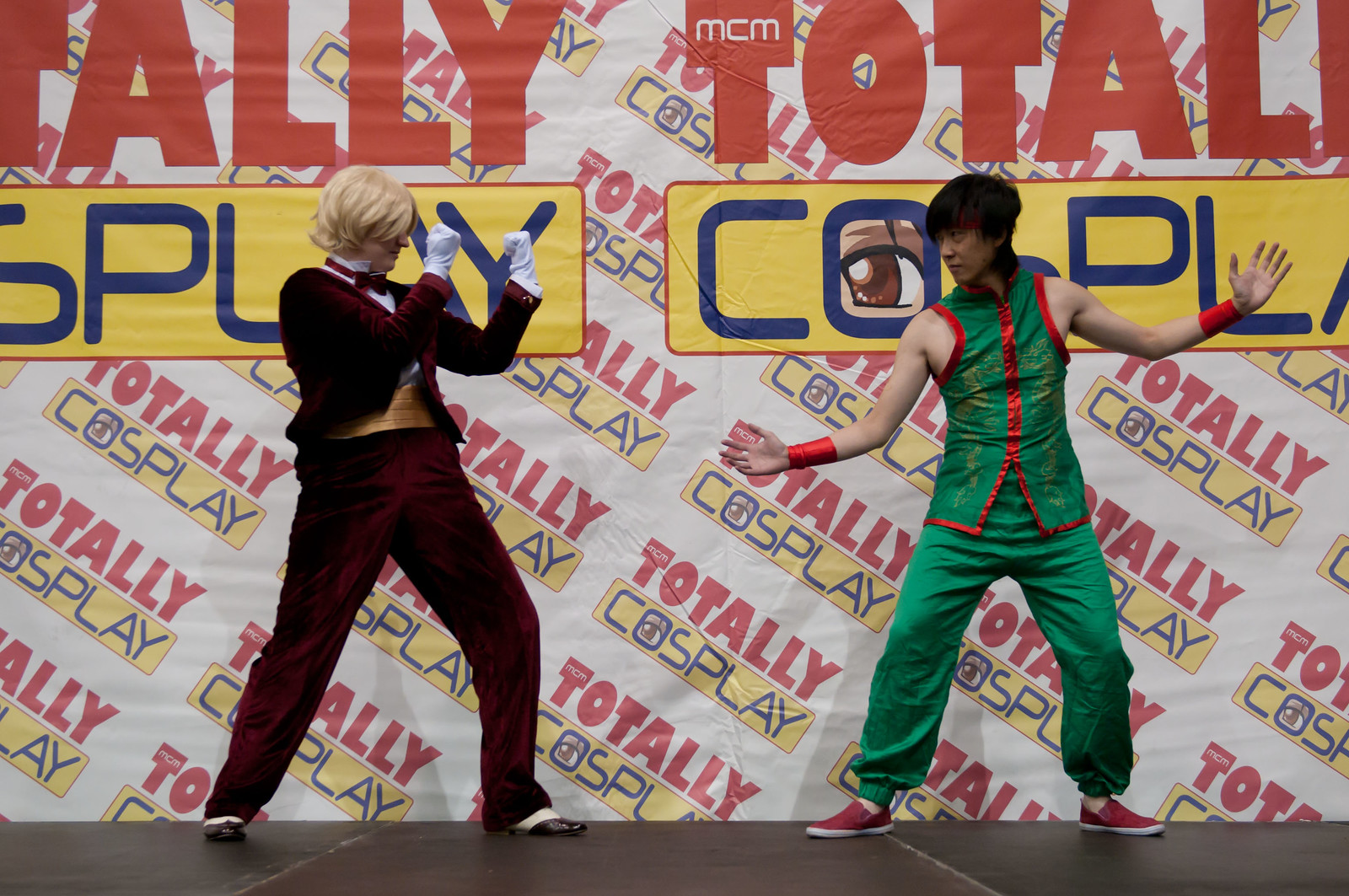In this vibrant image, two men are standing on a brown stage against a backdrop filled with repeating logos that read "Totally Cosplay" in alternating red and blue-yellow text, the word "Totally" highlighted in red and "Cosplay" in blue on a yellow background with an eye in the "O". The man on the left is dressed in a vivid red velvet suit, complete with matching pants, a white shirt, a colorful cummerbund in either green or gold, and a red bowtie. His ensemble is complemented by white gloves, and he strikes a classic fighting stance with his fists raised, channeling a vintage pugilistic vibe. He sports a blonde wig, enhancing his costume's period feel. The man on the right contrasts him with a more modern look, wearing a green sleeveless tunic edged in red trim, green pants, and red shoes. He accessorizes with red wristbands and has his black hair styled appropriately for his character. His pose, with one arm raised and the other slightly lowered, suggests he is ready for action, adding to the playful, competitive atmosphere. The scene captures the essence of a cosplay performance, with both men appearing poised for a mock battle reminiscent of Street Fighter or Mortal Kombat.